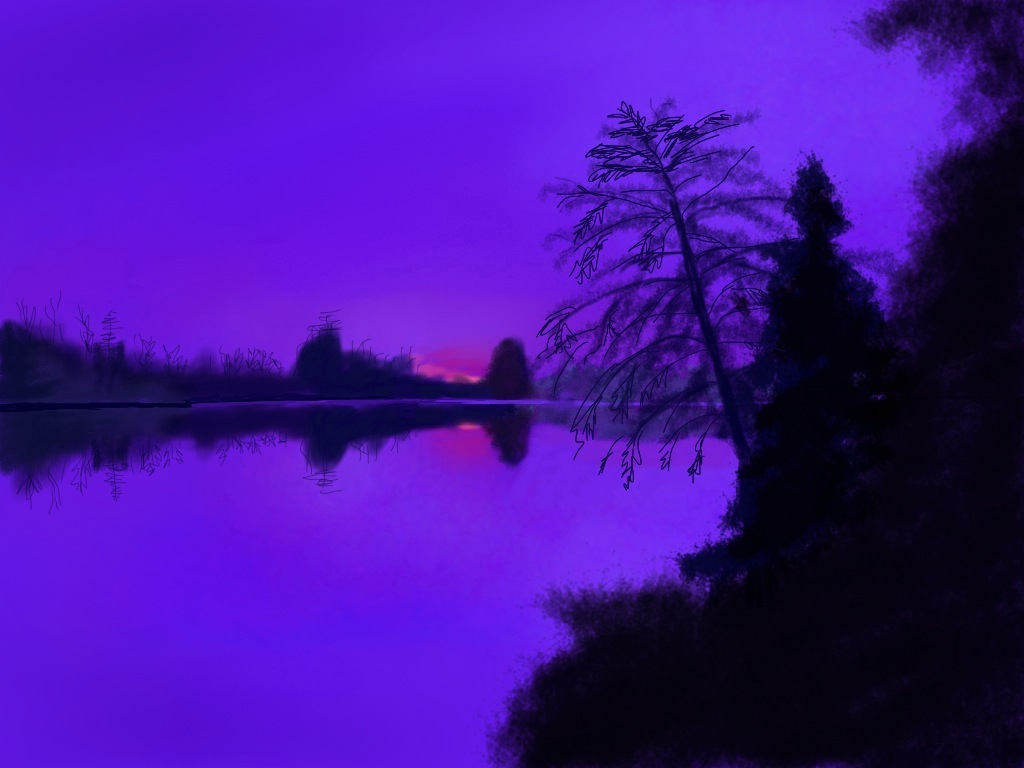This stunning photograph captures a mesmerizing moment during either sunrise or sunset when the sky transforms into an intense and vibrant shade of purple. The unique and surreal hues suggest significant artistic manipulation, enhancing the colors to create a view that is both breathtaking and otherworldly. The depth and brightness of the purple sky in this image present a spectacle that is rarely, if ever, seen in nature, evoking a sense of wonder and beauty that the photographer or artist yearned to depict.